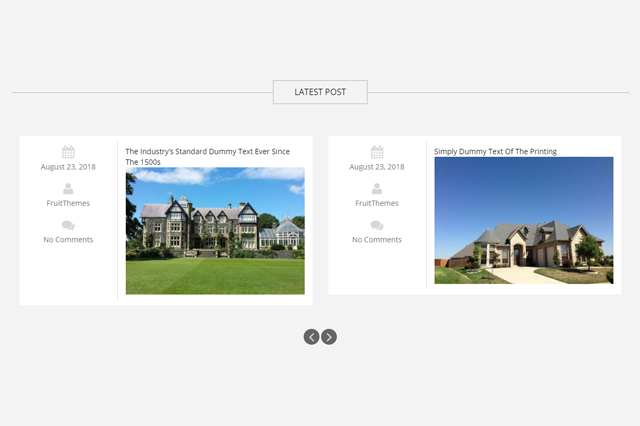The webpage features a clean, minimalist gray background. At the top, a rectangular box labeled "Latest Post" in a bold black font draws immediate attention. Below this header, two photographs are presented side-by-side.

The photograph on the left is framed by a pane on its left side, where a small calendar icon displays the date "August 25, 2018." Below the date, an icon representing a user account appears, followed by indistinct text, possibly "fruit themes" or something similar. Beneath this text, a comment icon indicates "No comments."

To the right of this pane, a bold black font headline reads, "Industry standard dummy text ever since the 1500s." Below this, the photo showcases a large, stately house, conveying a sense of grandeur.

The photograph on the right mirrors the left with the same arrangement: a calendar icon, user account icon, some text, and "No comments." Above this photo is a headline in a bold black font saying, "Simply dummy text of the pricing," although the font size is slightly smaller and harder to read. The photo depicts another house, different in style but equally notable.

Beneath these photos are two navigation buttons: a left-facing arrow ("<") for going back and a right-facing arrow (">") for moving forward.